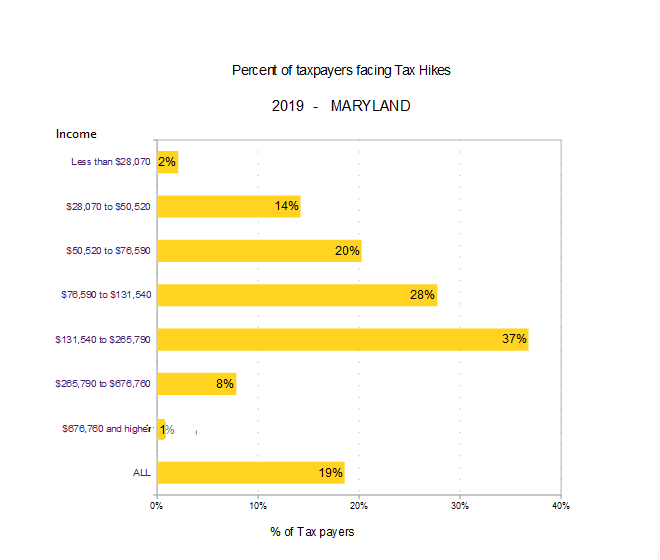The image showcases a detailed bar graph under the title "Percent of Taxpayers Facing Tax Hikes, 2019, Maryland." The graph, set against a white background, has a vertical axis labeled with income brackets ranging from "Less than $28,070" to "676,780 and higher." On the horizontal axis, percentages from 0% to 40% are listed with the label "Percent of Taxpayers" beneath it. 

Each income bracket is represented by a yellow bar indicating the percent of taxpayers facing tax hikes:
- Less than $28,070: 2%
- $28,070 to $50,520: 14%
- $50,520 to $76,590: 20%
- $76,590 to $131,540: 28%
- $131,540 to $265,790: 37%
- $265,790 to $676,780: 8%
- $676,780 and higher: 1%
- All (combined category): 19%

The standout feature is the bar for the income bracket $131,540 to $265,790, which is the longest at 37%, indicating it has the highest proportion of taxpayers facing tax hikes. Other key details include a significant drop in percentage to 8% for the next income group, with an overall percentage range visible from left to right at the bottom of the graph.